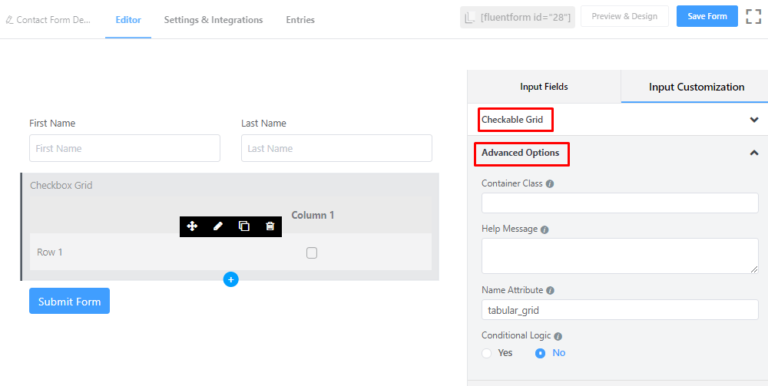The image showcases a customizable contact form interface with multiple input fields. The form includes sections for users to input their first name and last name. A notable feature is the "Check Grid" box presented within a gray column. Adjacent to the form fields, on the right side, there is a blue plus sign and a "Submit" button. The form allows users to customize input fields according to their preferences, a functionality highlighted by the label "Input Fields Input Customization." Additionally, there are various elements within the form, marked by red boxes, including "Check Grid Advanced Options," "Container Glass," "Help Message," "Name Attribute," and "Condition." The "Condition" field provides a yes/no option, which, in this instance, is indicated as 'no.'